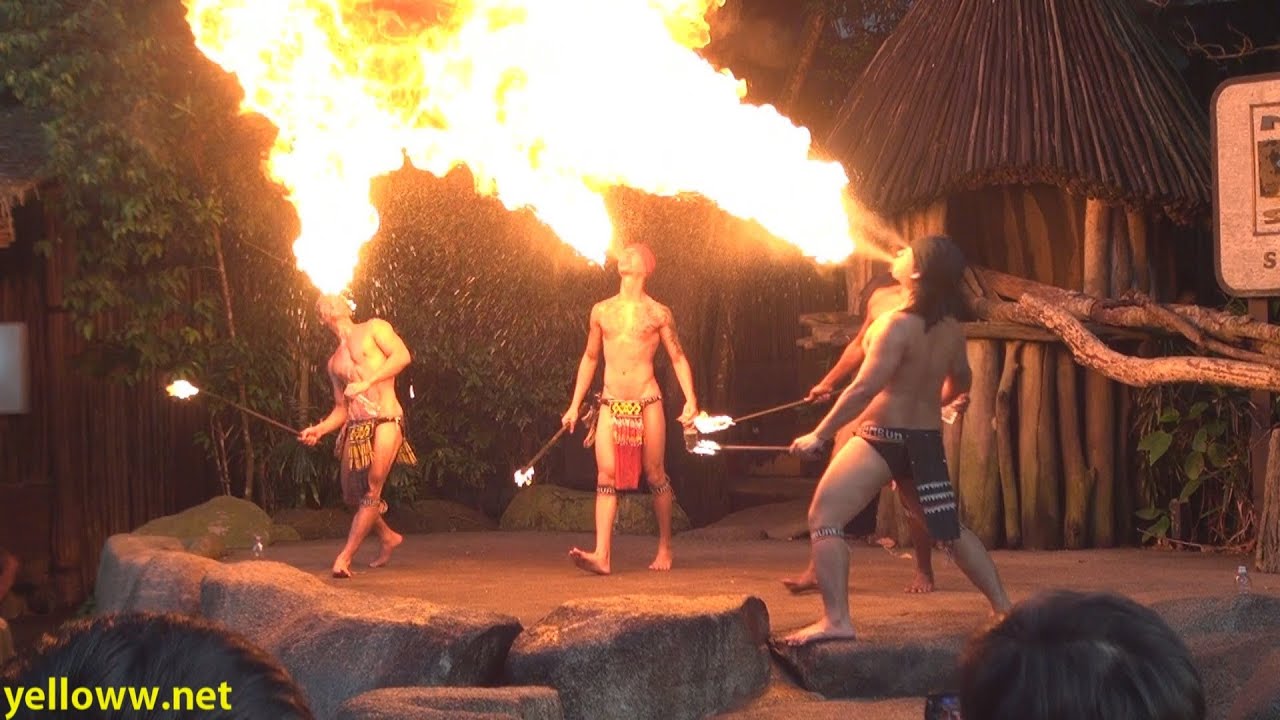In this computer-generated nighttime image, four Polynesian-themed fire breathers, dressed in colorful loincloths, stand on a stone stage with boulders outlining it. Each man is shirtless, holding a lit torch, and simultaneously exhaling large plumes of fire. They are arranged in a semi-circle, creating a striking visual as their flames merge into a massive fireball above them. The stage is set against a lush tropical backdrop, including green vines, a straw-thatched tiki hut, and various branches. Audience heads are visible in the foreground, indicating a live performance. The image features yellow text at the bottom left corner that reads "YELLOWWW.NET".